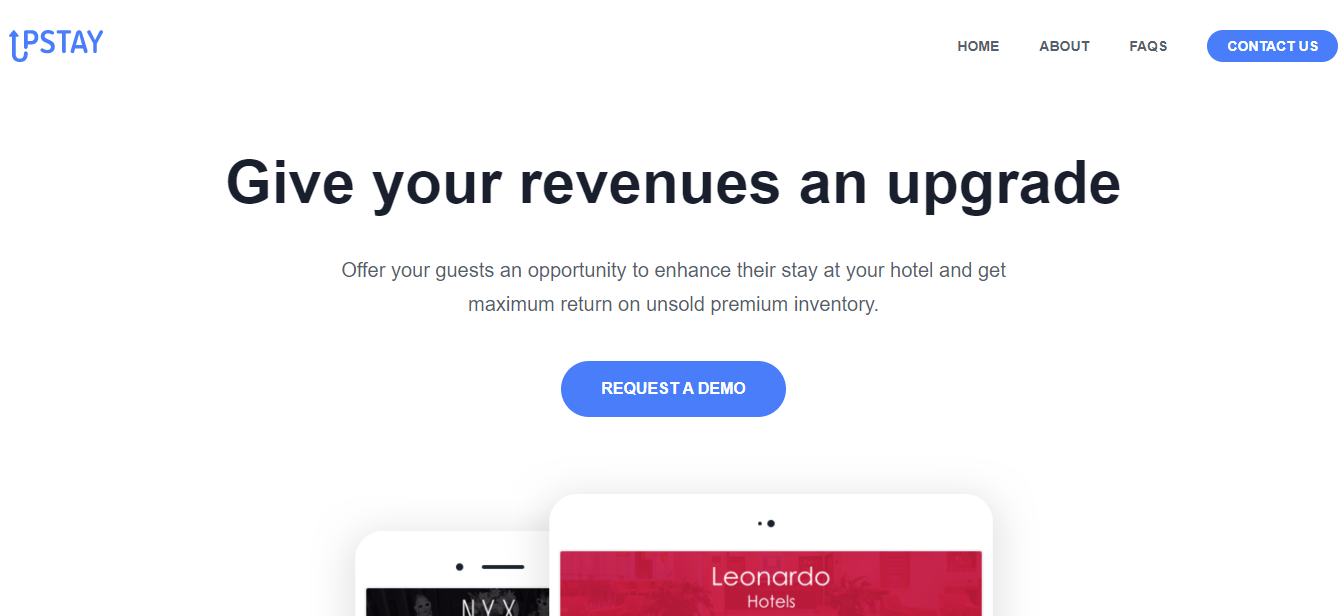**Screenshot of the Upstay Website**

In this screenshot of the Upstay website, the company's logo is prominently placed in the top left corner. The logo features a blue arrow, creatively integrating the letters 'U' and 'P,' with the arrow descending from the 'P,' arching below, and pointing back upwards. The background of the website is clean and white, giving it a modern and uncluttered appearance. 

The site header includes navigation links to the "Home," "About," "Frequently Asked Questions," and "Contact Us" pages. The central heading of the site reads "Give Your Revenues an Upgrade," emphasizing their core mission. Below this main heading is a subheading that elaborates on the service offered: "Offer your guests an opportunity to enhance their stay at your hotel and get maximum return on unsold premium inventory."

A prominently placed button beneath the subheading invites visitors to "Request a Demo." Following this call to action, there is a visual mockup showcasing the service in action. On the left is an image of a cell phone displaying the NYX Hotel interface, and on the right, a tablet displays the Leonardo Hotels interface. Both devices suggest the integration of Upstay’s service with hotel management systems. The overall presentation indicates that Upstay offers a hotel stay upgrade service designed to maximize revenue from unsold premium inventory.